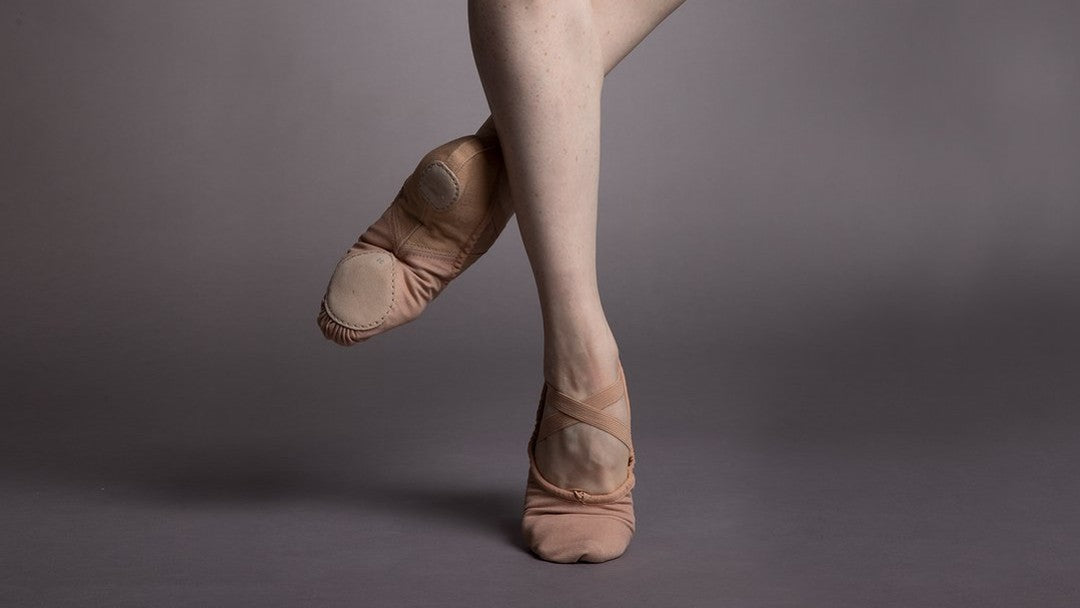The image is a horizontally aligned, rectangular photograph with a background that transitions from medium gray at the top, to darker gray in the middle, and back to medium gray at the bottom, giving the impression of a shadow. In the center of the image are the legs of a ballerina, depicted from just below the knees down to her feet. She is wearing light brown, or flesh-colored ballet slippers with cross straps over the top. One foot is prominently featured on the ground, on pointe, with the arch fully extended, while the other leg is bent behind it, crossing over and showing the bottom of its slipper. The visible sole of the raised foot has a suede-like texture and there are detailed wrinkles in the fabric of the slipper, highlighting the realism of this elegant pose. The dancer's toe-down foot faces directly towards the viewer, and the overall setting feels as though it could be indoors, emphasizing the detailed and expressive nature of her ballet position against the subtly blended gray background.